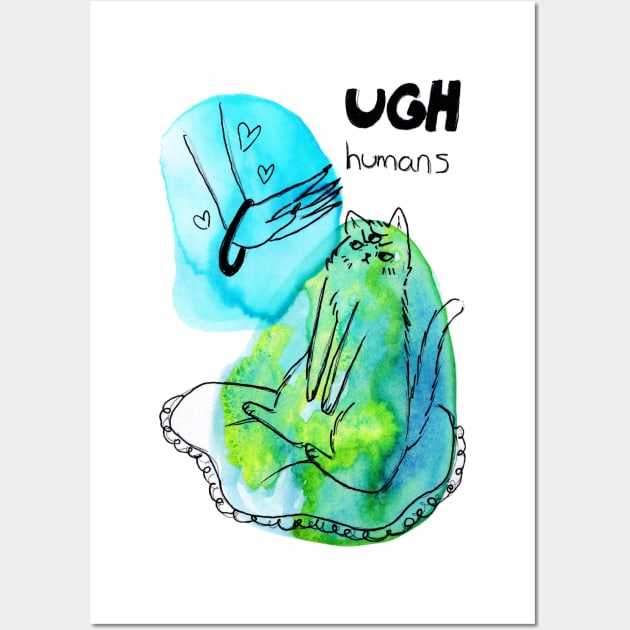In this colorful and playful comic-style painting, we see a detailed scene of a cat sitting on a cushion, rendered in shades of blue and green. The cat looks visibly annoyed, staring up at a human hand that hovers just above it, adorned with a black bangle and surrounded by small heart-shaped drawings, illustrating the human's affection. The hand, depicted in a line drawing, appears to be frozen mid-reach, emanating from a blue, circular splotch, further emphasizing its motion. Above the cat and to the upper right of the hovering hand, bold black text reads "UGH," followed by "humans" in smaller letters, capturing the cat's exasperated sentiment. The entire scene is set on a rectangular white sheet, with blue and green colors creatively painted within and around the elements, encapsulating the humorous dynamic between the feline and human characters.